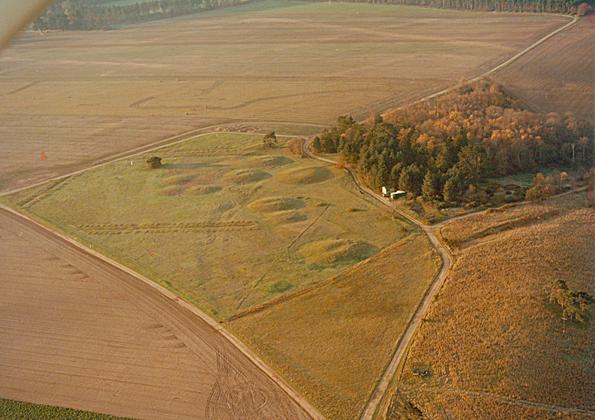The aerial image reveals a vast, arid landscape marked by clearly defined sections and dirt roads crisscrossing through the terrain. At the center of the photo, a trapezoidal field, tilted about 45 degrees to the right, stands out with several circular mounds adorned by depressions in their centers, resembling Indian burial grounds. This field is partially green while the surrounding areas are largely brown or bare dirt. To the center-right of the image, a significant cluster of trees contrasts with the otherwise sparse landscape. This greener area, featuring a mix of fully-leaved and autumn-turning trees, contains a small section of water and two parked vehicles, possibly trailers. Beyond this cluster and across the open expanse, another line of trees delineates the horizon, lining a distant road. Additionally, the top-left corner of the image subtly captures what appears to be the wing of an airplane, hinting at the aerial vantage point from which this photograph was taken.